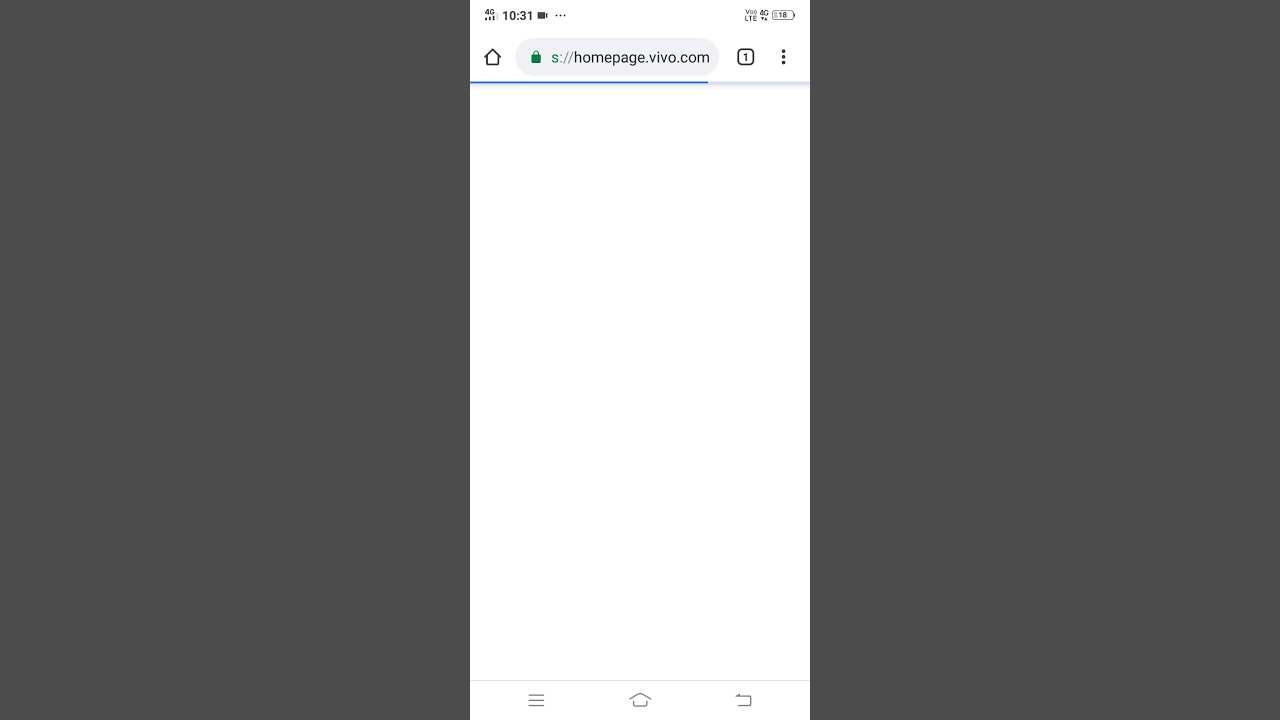The image displays a smartphone screen with a gray rectangular status bar at the top, showing the time as 10:31, a battery level at 18%, and a 4G network indicator. The browser is open to the website homepage.vivo.com, using a secure HTTPS connection as indicated by the preceding 'https://'. Within the user interface of the browser tab, there is a home icon, a square symbol labeled with the number '1', and three vertical dots which likely represent additional options or settings. At the bottom of the screen, there are several gray icons including a hamburger menu (three horizontal lines), another home icon, and an icon resembling a clockwise arrow suggesting a refresh or reload function, characterized by a partial square shape starting from the bottom, moving right, then up, and curving back to the left with an arrowhead at the end.